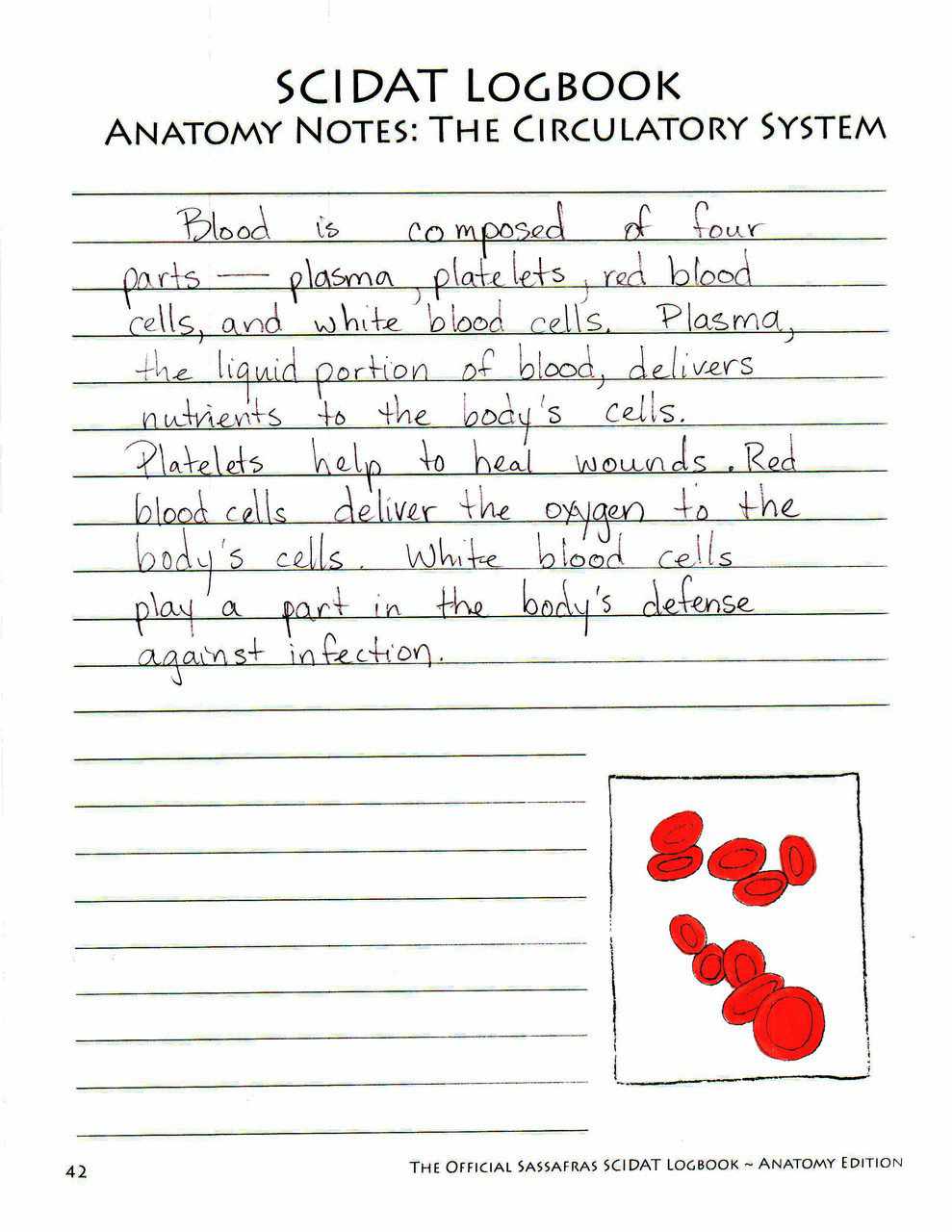The image depicts a notebook page with ruled lines, featuring a heading in capital letters that reads, "SciDAD Logbook, Anatomy Notes, The Circulatory System." Below the heading, the handwritten notes explain: "Blood is composed of four parts: plasma, platelets, red blood cells, and white blood cells. Plasma, the liquid portion of blood, delivers nutrients to the body's cells. Platelets help to heal wounds. Red blood cells deliver oxygen to the body's cells. White blood cells play a part in the body's defense against infection." In the bottom right corner, there is an inset of red blood cells, depicted as oval-shaped structures. At the very bottom, a footnote states, "The official SAS FRS SciDAD Logbook, Anatomy Edition." The page number, 42, is visible in the left corner of the image. The page looks very much like typical notebook paper, enhancing its academic feel.